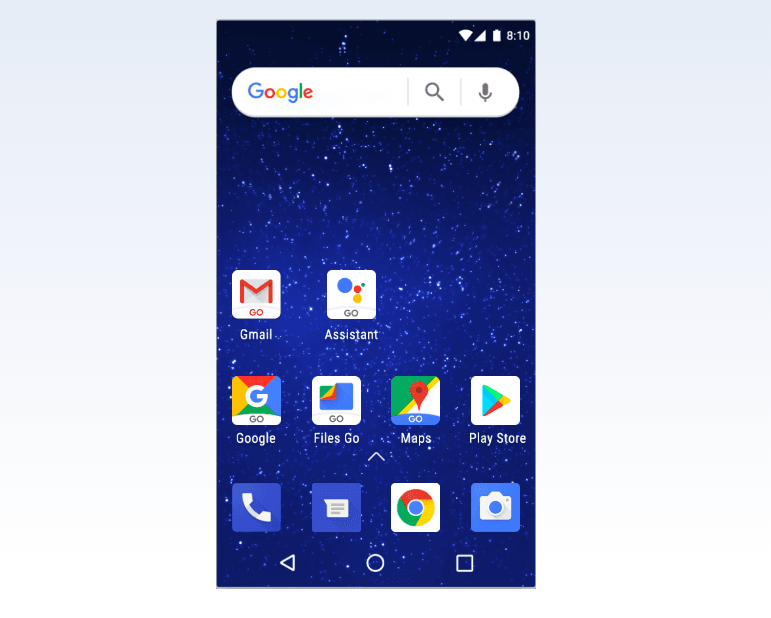The image showcases the front view of a cell phone screen. The screen displays the time as 8:10 and indicates a strong network connection. At the top of the screen is a white oval search bar that prominently features the word "Google" in the brand's signature colors: red, blue, yellow, and green. This search bar also includes a search icon and a microphone symbol.

The screensaver is particularly eye-catching, depicting a nighttime scene that transitions from a deep black at the top to a lighter, purplish-blue hue towards the bottom. Scattered throughout this gradient are numerous white dots resembling stars, adding to the serene, celestial aesthetic.

Below the search bar, various app icons are arranged neatly. The Gmail icon stands out with a bold "M." The Google Assistant app, labeled "Go," is displayed with colored bubbles in blue, yellow, green, and red. The Google Go app is also present, featuring the same Google brand colors. Other icons include Files Go, Maps Go (marked by a red location pin), and the Play Store, all adorned in the Google's colors.

Additionally, there are several standard icons: a blue phone icon, a blue messaging icon, a white Google Chrome icon, and a blue camera icon. These icons appear to be a consistent feature at the bottom of the screen, typical of most cell phones.